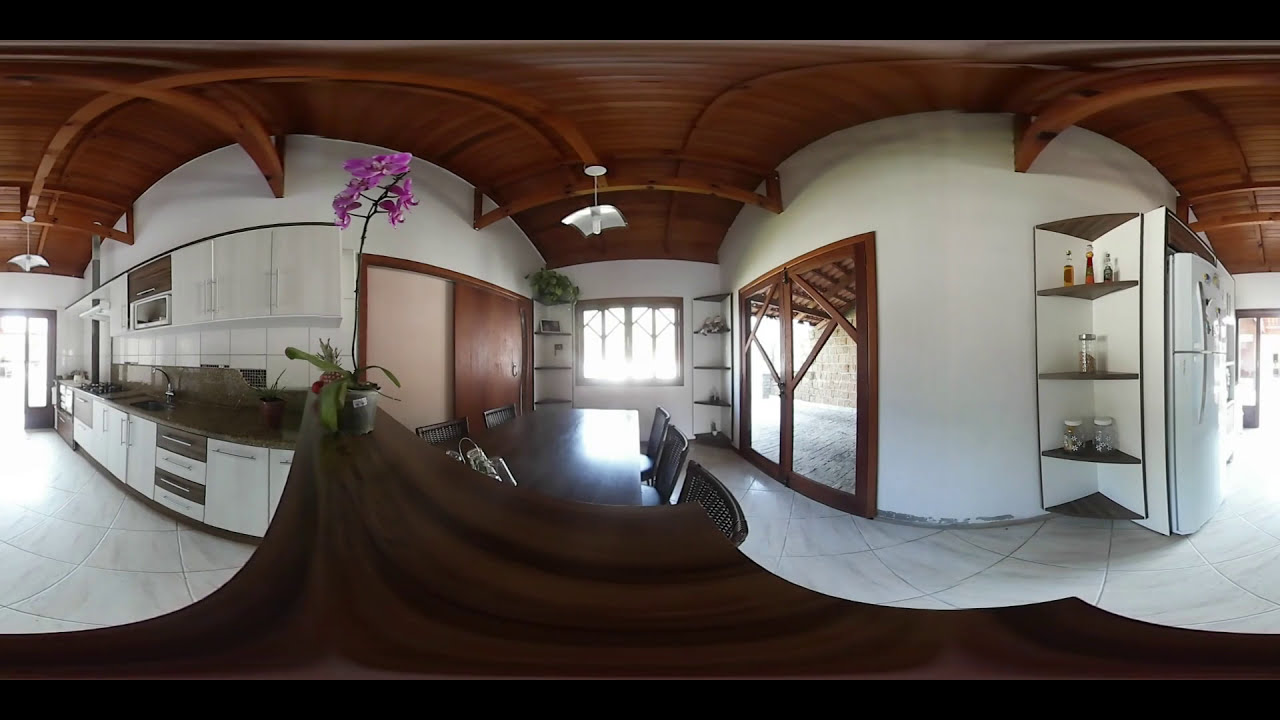The image captures a 360-degree view of a modern kitchen and dining area, characterized by a cohesive white and black color scheme accented with dark wooden trim. The focal point on the right side of the image is the kitchen, showcasing sleek white cabinets with thin silver handles and a contrasting dark gray or black countertop. Notable fixtures include a silver microwave positioned above the sink, a sleek modern white fridge adorned with magnets, and various kitchen appliances and utensils.

The kitchen floor features white tiles, enhancing the room's clean aesthetic. A central breakfast bar, finished in dark wood, houses a potted orchid with delicate pinkish-whitish flowers.

In the middle of the image is a spacious dining area anchored by a rectangular dark brown wooden table surrounded by six chairs—three on the right and two on the left. The table is set with pots and utensils, echoing the kitchen's practical yet stylish theme. The backdrop includes doorways leading to other rooms and a large window with geometric square and triangular frames, further illuminating the space.

From the ceiling, a light fixture hangs, highlighting the rustic charm of the darker wooden roof. Near the window, glass doors open to reveal an outdoor area, inviting a seamless transition between indoor and outdoor living. Additionally, a corner stand in the room displays jars and glass bottles, adding to the room's organized yet homely feel.